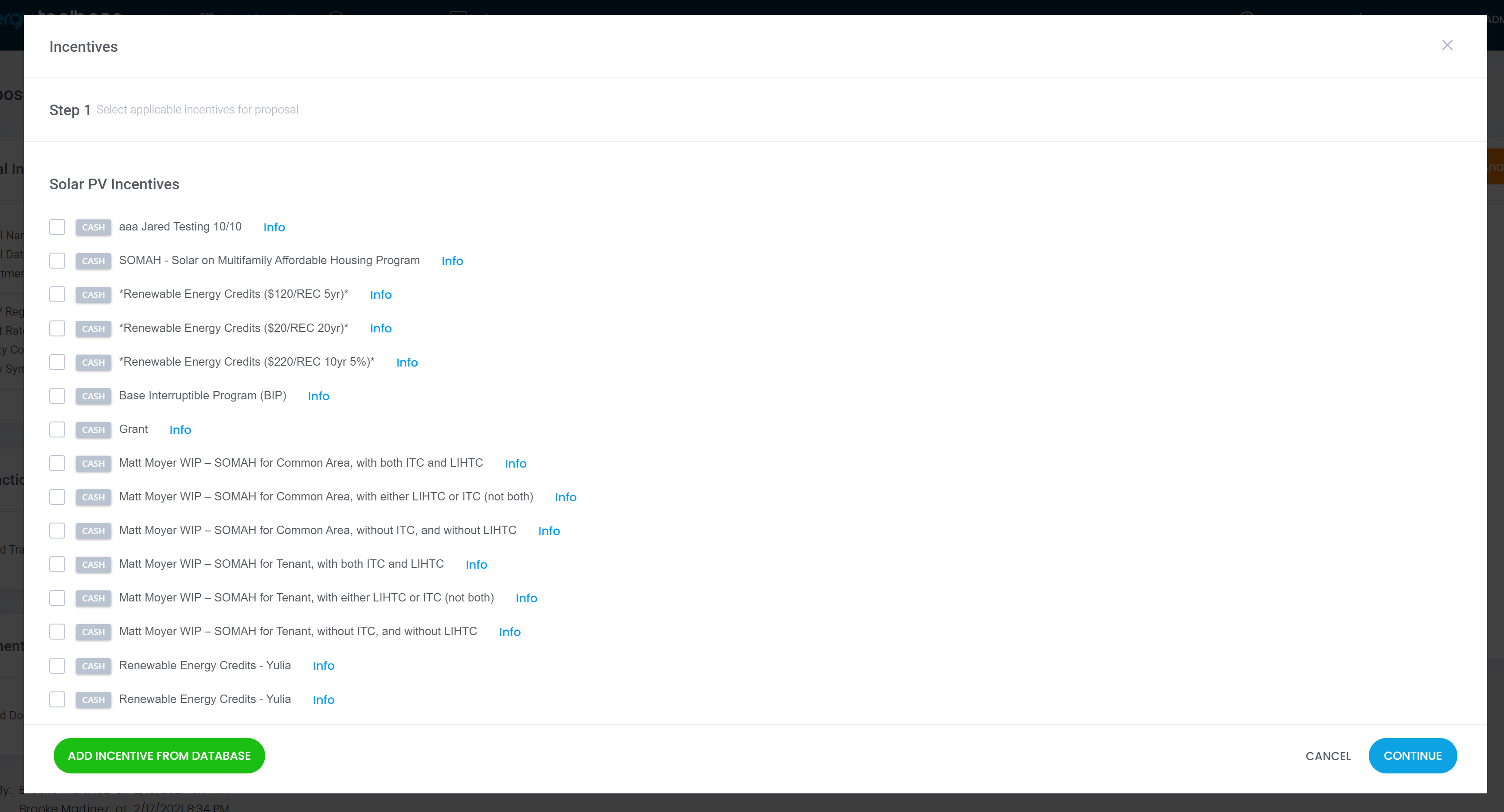The image depicts a web page interrupted by a prominent white pop-up box, which obscures the underlying content. In the top left corner of the pop-up box, the word "Incentives" is written in black text. The top right corner features a gray "X" icon, allowing users to close the pop-up. Within the pop-up, "Step 1" is indicated, followed by small gray text that reads "Select Proposal." Below this, in bold black text, the phrase "Solar PV Incentives" is displayed. 

The pop-up lists multiple items, each accompanied by a check box and a gray button labeled "Cash." Additionally, blue hyperlinks are provided beside each option for more details; one of these hyperlinks is labeled "Reversible Energy Credit," and another indicates a grant. At the bottom of the pop-up, there is an option labeled "Add Incentives from Database" and a prominent green button, likely for finalizing the selections or moving to the next step in the process.